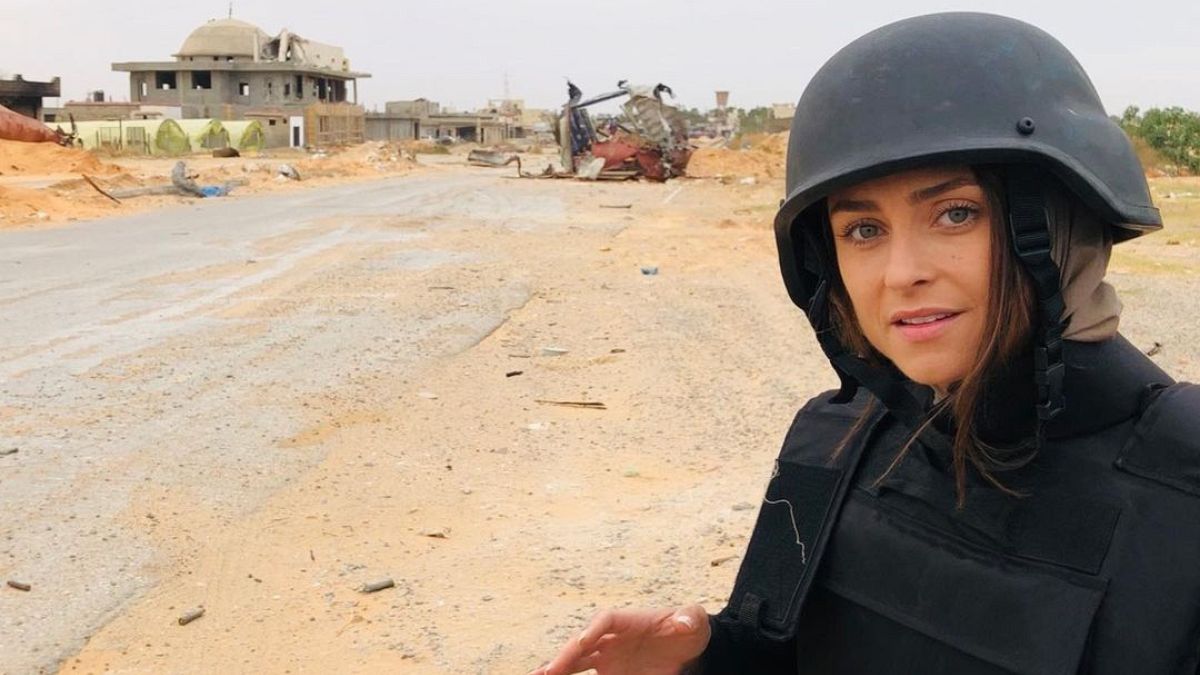The image captures a woman of lighter skin complexion standing outdoors in a large dirt area. She is dressed in black tactical gear, including a black jacket, a bulletproof vest, and a black military-style helmet, under which a taupe head covering can be seen, with her brown hair spilling out. The woman, with blue eyes, is looking directly at the camera and gesticulating with her right hand. Positioned on the right side of the rectangular, horizontally oriented photo, she stands in front of a barren dirt path. The background reveals a combination of mangled machinery and a gray stone building that appears to be either under construction or in a state of demolition. The structure has a basilica-like top and is hollowed out. Additionally, a road flanked by sand or dirt, a partially visible home, and green trees can be seen. The sky is gray, and the setting is well-lit with natural daylight, enhancing the photo's clarity. No other people are present, and there are no words or numbers in the image.